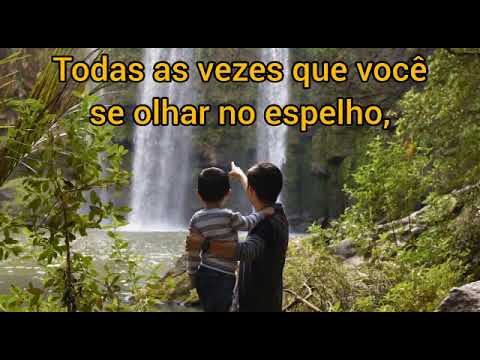In this image, we observe a young man and a child standing on a green, vegetation-rich shore, both with their backs turned to the camera. The scene is filled with lush greenery, including small trees and vines, along with some visible rocks. In the distance, a waterfall cascades into a small body of water, which appears to be the beginning of a river.

The child, who has dark hair, is wearing a striped shirt and pants, placing his right hand on the man's shoulder. The man, likely the child's father, is on the right, pointing towards the distant waterfall with his right hand, while his left arm is wrapped around the boy. He is dressed in a dark-colored shirt and a wristwatch. Both figures are standing close to the water's edge amidst the surrounding foliage.

Prominently displayed across the middle of the image is yellow text outlined in black, in Portuguese. It reads: "Todas as vezes que você se olhar no espelho," which translates to "Every time you look in the mirror." This appears to be a screen grab from a video, adding a poignant message to the serene, nature-filled scene.